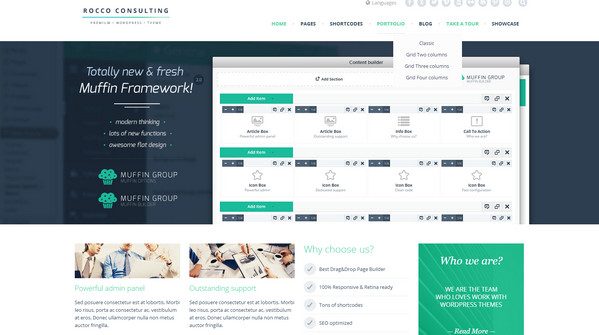This is a detailed description of a web page from Rocco Consulting, featuring a long, horizontal layout. On the left side against a dark blue background with two different shades of blue, there is a prominent header stating "Totally New and Fresh Muffin Framework." Below this header are three bullet points: "Modern Thinking," "Lots of New Functions," and an illegible first word followed by "Flat Design," which might say "Awesome Flat Design."

At the bottom left, there are two Muffin Group logos stacked vertically, each accompanied by the name "Muffin Group." To the right side of the page, there is a series of boxes with some containing green buttons with white text and others featuring black and white designs. The text within these boxes is too small to read clearly.

The page is currently open to one of seven tabs located at the top of the page. Three of these tabs are in yellow-green, and the remaining are in black. The tab labeled "Blog" is currently selected, revealing four different choices that are too small to decipher. Below these tabs are two menu choices accompanied by stock business photos. The first photo, topped with a green headline, is titled "Powerful Admin Panel." The second photo to the right, also with a green headline, is titled "Outstanding Support," each with a paragraph of text beneath them.

To the right of these photos, there is a "Why Choose Us" box outlining four reasons to choose Rocco Consulting, including "Tons of Shortcodes" and "SEO Optimized." At the bottom right of the image, there is a green box with white text that says, "Who We Are: We are the team who loves working with WordPress."